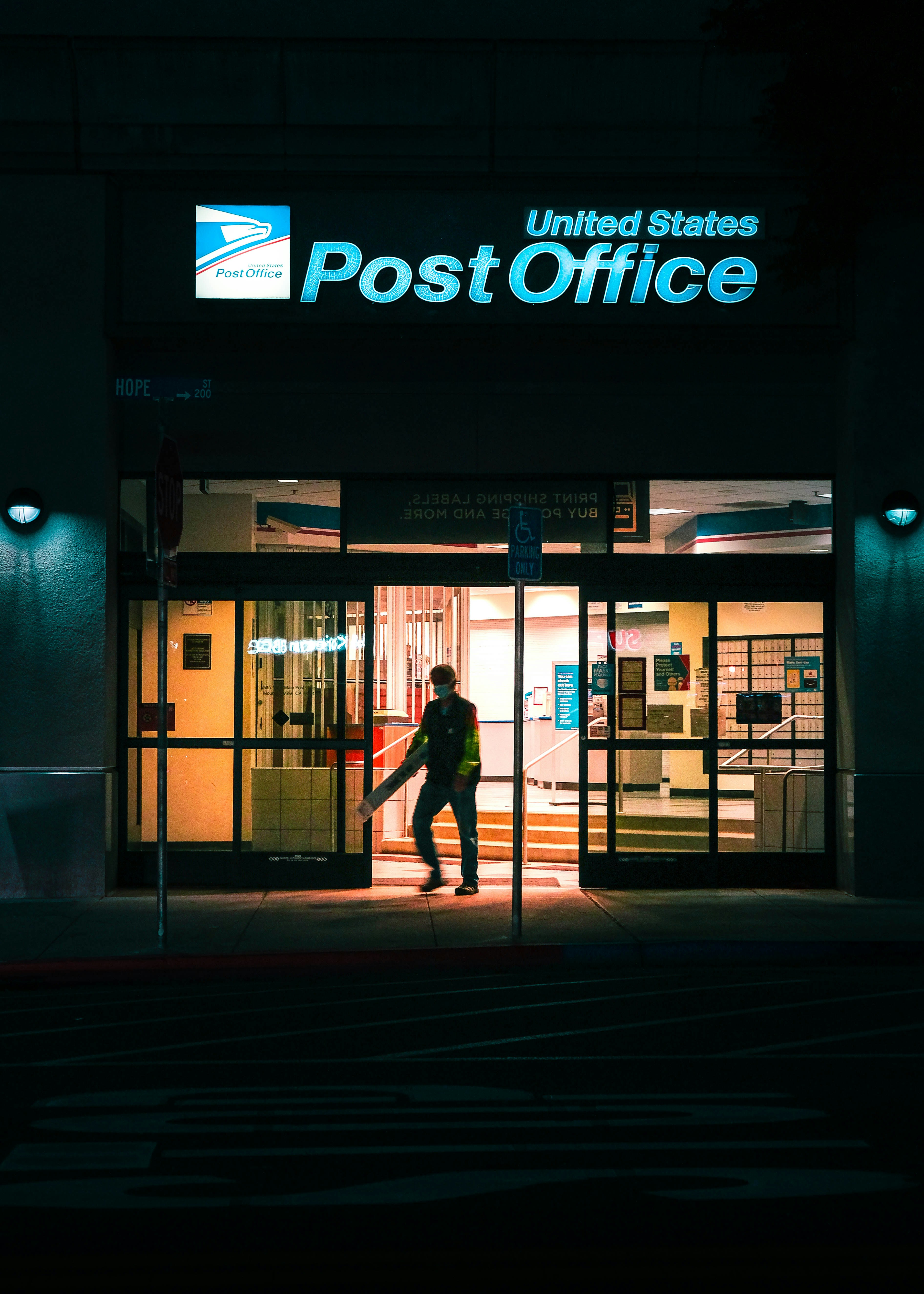The photograph captures the outside of a United States Post Office at nighttime. The large, illuminated blue text "United States Post Office" and the corresponding USPS logo (featuring an eagle) are prominently displayed at the top of the building. Below the glowing sign, the building has glass sliding doors which are open, and a person, whose silhouette is barely distinguishable due to the dark setting, appears to be exiting. This individual is wearing a blue face mask and carrying a long package as they walk towards the left side of the frame.

The scene around the building includes a well-lit parking space with a prominently displayed handicap parking sign. Additionally, there is a similar sign nearby indicating the location, possibly reading "Hope Street." Outside, on either side of the glass doors, wall-mounted lights cast a soft glow on the grey walls, partially illuminating the parking area and the sidewalk in front of the building. Inside the post office, the bright yellow lights reveal a reception desk, a stairway leading to post boxes for mail collection, and various posters adorning the interior walls.